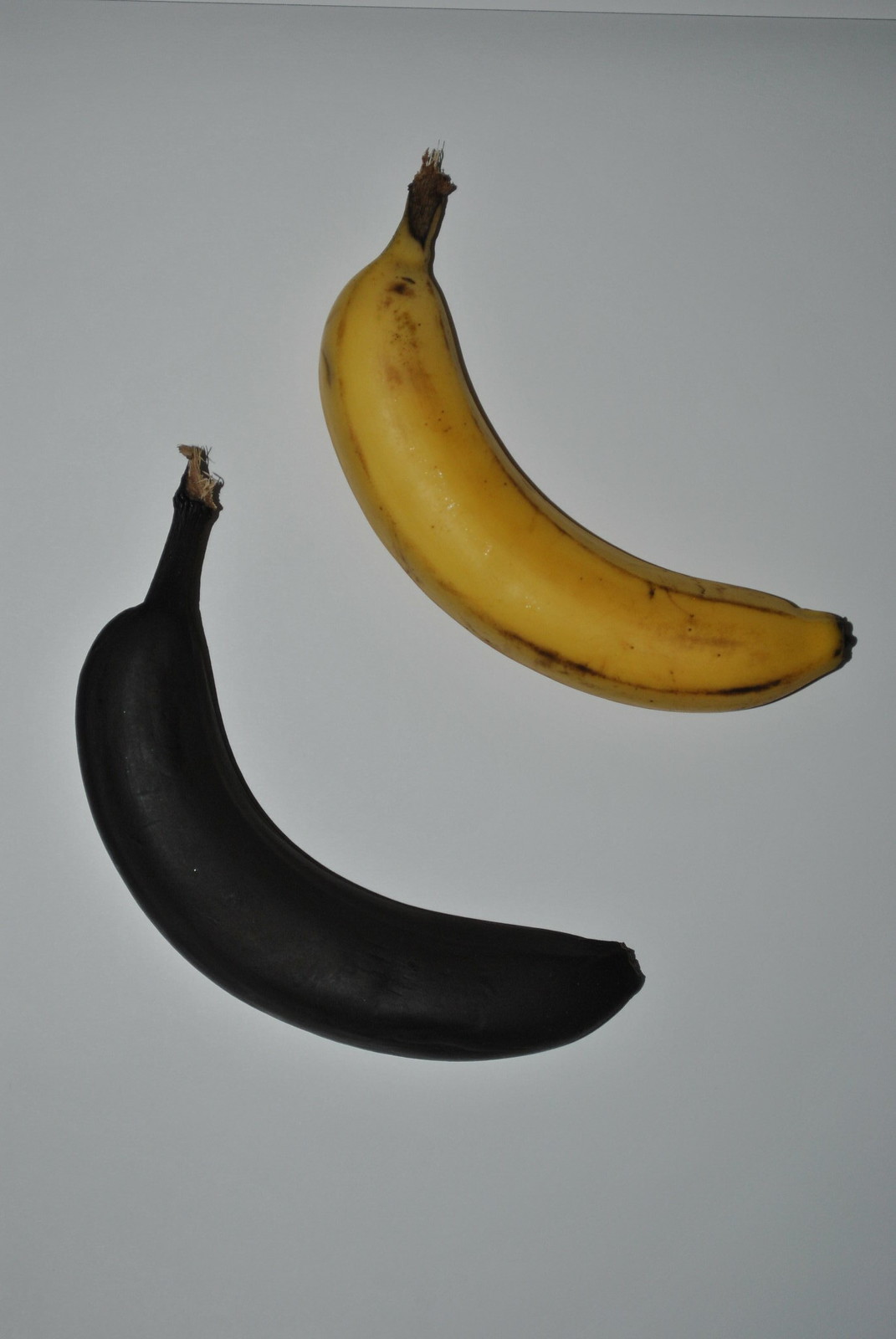The image features two bananas placed on a muted, greyish-white background. The banana positioned slightly to the top right is a ripe, yellow banana with small brown specks, typical of natural ripening. It has the characteristic tuft at the end where it was separated from the bunch, as well as the smaller tips at the bottom. The second banana, situated at the bottom left, appears to be painted or sprayed jet black, lacking the usual details of over-ripening such as discoloration or shriveling. This banana retains the same shape and size as the yellow one, suggesting it has not undergone any decay. The only variation in its color is at the point where it was torn from the bunch, revealing a brownish-beige hue with visible fibers. Together, these bananas provide an intriguing contrast of natural ripening versus artificial coloring.